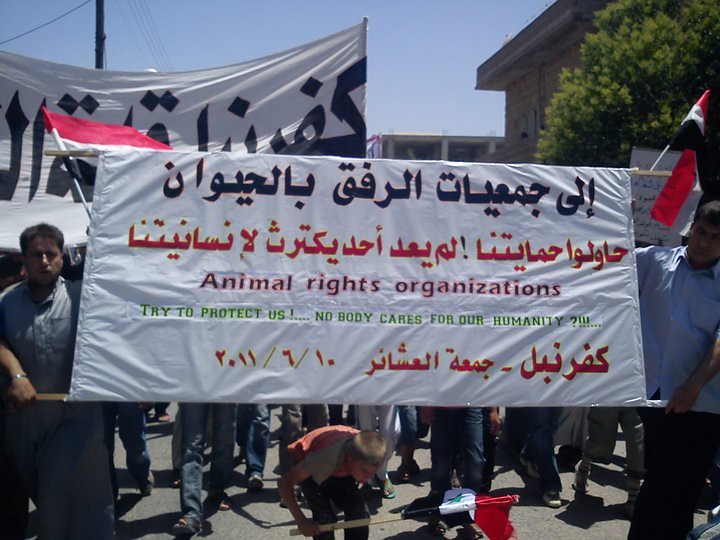In this color photograph, an outdoor event that appears to be a protest is captured in vivid detail. At the forefront, two men are holding up a large white banner, which is suspended between two long metal rods, approximately 10 feet each. The banner features multiple lines of text: at the top, there is a row of bold black text in a language that appears to be from the Middle East, likely Arabic, with elements indicating the Iraqi flag. Below that, in red text, more text is followed by English phrases in black and green that read, “Animal rights organizations” and “Try to protect us. Nobody cares for our humanity.” The bottom of the banner includes additional red text in the same unidentified language. 

Beneath the banner, a young boy is seen holding a flag. Surrounding the banner, there is a crowd of people also holding flags amidst the asphalt pavement and visible power lines above them. Behind the main banner, to the left, another large banner with bold black text on a white background is present. The background is punctuated by a few green trees, some buildings, and a clear blue sky, adding to the ambient context of the protest scene.